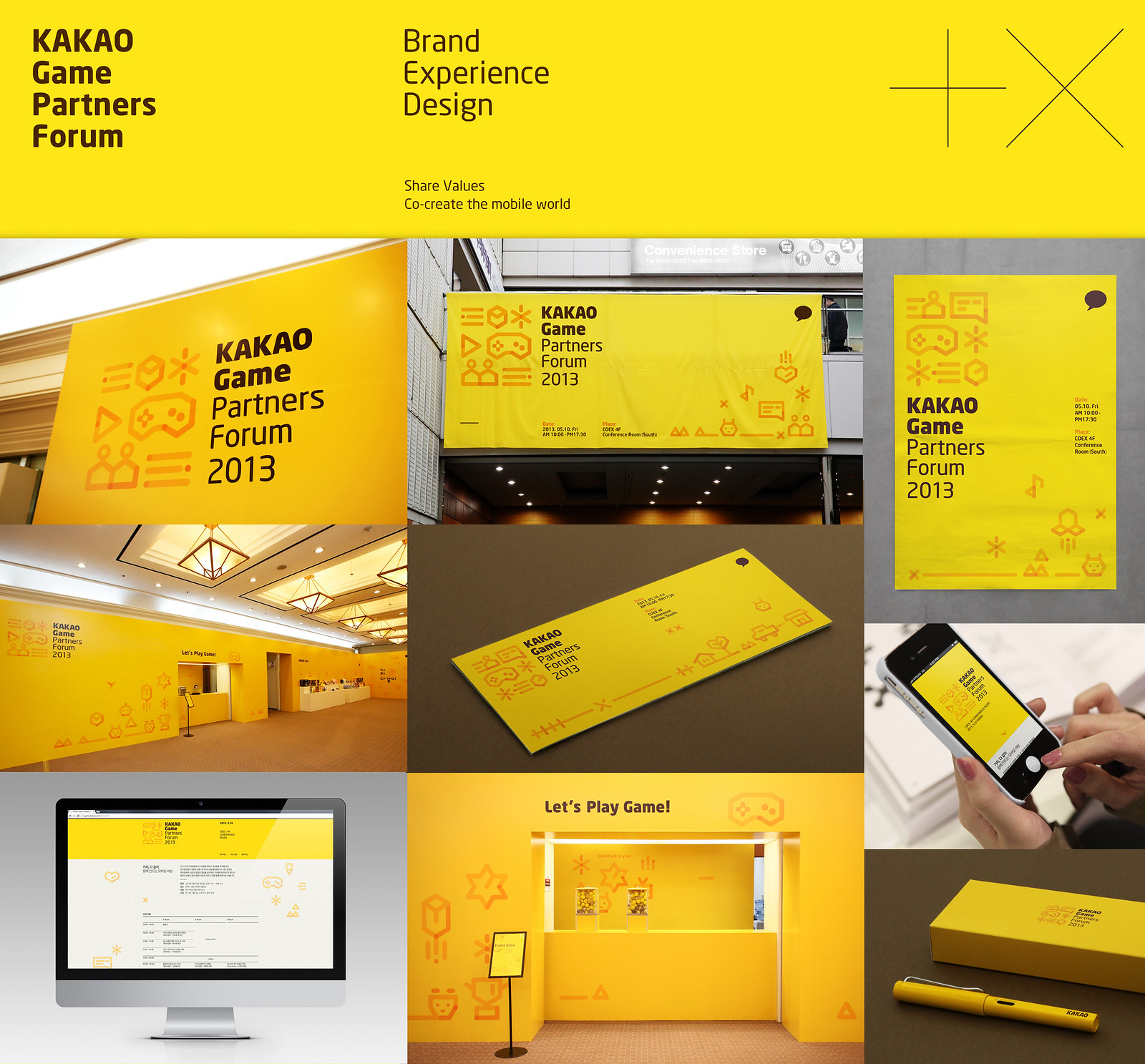The image comprises a 3x3 grid of smaller images, all centered around the theme of the Kakao Game Partners Forum, with a vibrant yellow background at the top that reads "Kakao Game Partners Forum" and "Brand Experience Design" in black text. The overarching theme is reinforced with a tagline emphasizing the forum's mission to "share values and co-create the mobile world." Each of the nine images showcases the forum's branding, represented through a sleek, almost cartoonish, yellow logo featuring a game pad, a person, and a message icon. This logo appears in various applications: on a large poster board within a room, a smaller yellow poster, an envelope, a phone held in someone's hand, and a yellow pen in a box. The consistent yellow hue ties the visuals together, making the branding unmistakable and cohesive. One image also features a plus sign and an X as part of the design elements. The logo is seen on a computer screen, emphasizing its versatile use across different mediums, reinforcing the brand's presence and identity from Kakao Game Partners Forum 2013.